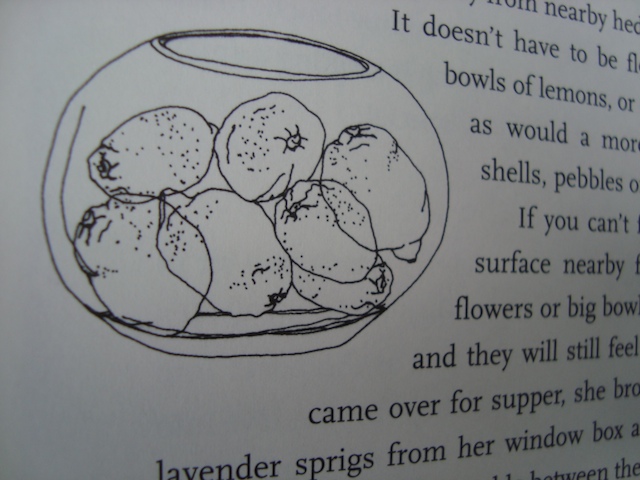The image is a highly detailed, close-up illustration on the page of a book or piece of paper. Central to the composition is a clear glass bowl, rendered in fine black lines, containing various types of fruit, including what appear to be six circular fruits, possibly pears, marked with black dots. The bowl is positioned slightly off-center, towards the top left of the page. Surrounding the bowl on the right side is black text that wraps around the illustration, though much of it is cut off and thus incomplete. Legible segments of the text include phrases like "it does have to be," "bowls of lemons," and "shells, pebbles," among others, hinting at a larger narrative that is mostly obscured. The background of the page is stark white with some subtle shadowing on the right side, enhancing the focus on the central illustration and text. The entire scene is well-lit and sharply in focus, emphasizing the intricate details and simplicity of the black and white palette.